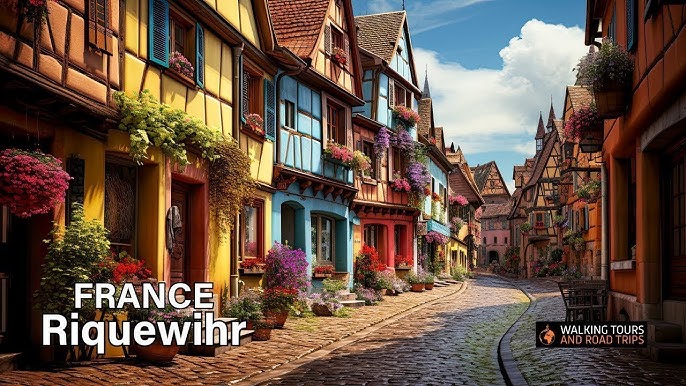This image captures a picturesque scene of Riquewihr, France, framed by a brightly sunny sky with a few clouds. A winding cobblestone street cuts through the center, bordered by vividly colored buildings. On the left, small houses painted in charming hues of yellow, brown, blue, and red each feature an array of plants adorning doorways, window frames, and hanging from the tops of door frames, showcasing flowers in green, white, purple, and red. The right side appears to host shops with similar plant life and outdoor tables and chairs adding to the quaint ambiance. A slight curb lines the street, enhancing the quaint feel of the village. In white text, the bottom left corner identifies the location as "France, Riquewihr," while the bottom right corner bears a small block of text on a black background with an image of the globe, stating "Walking Tours" and "Road Trip" in beige.